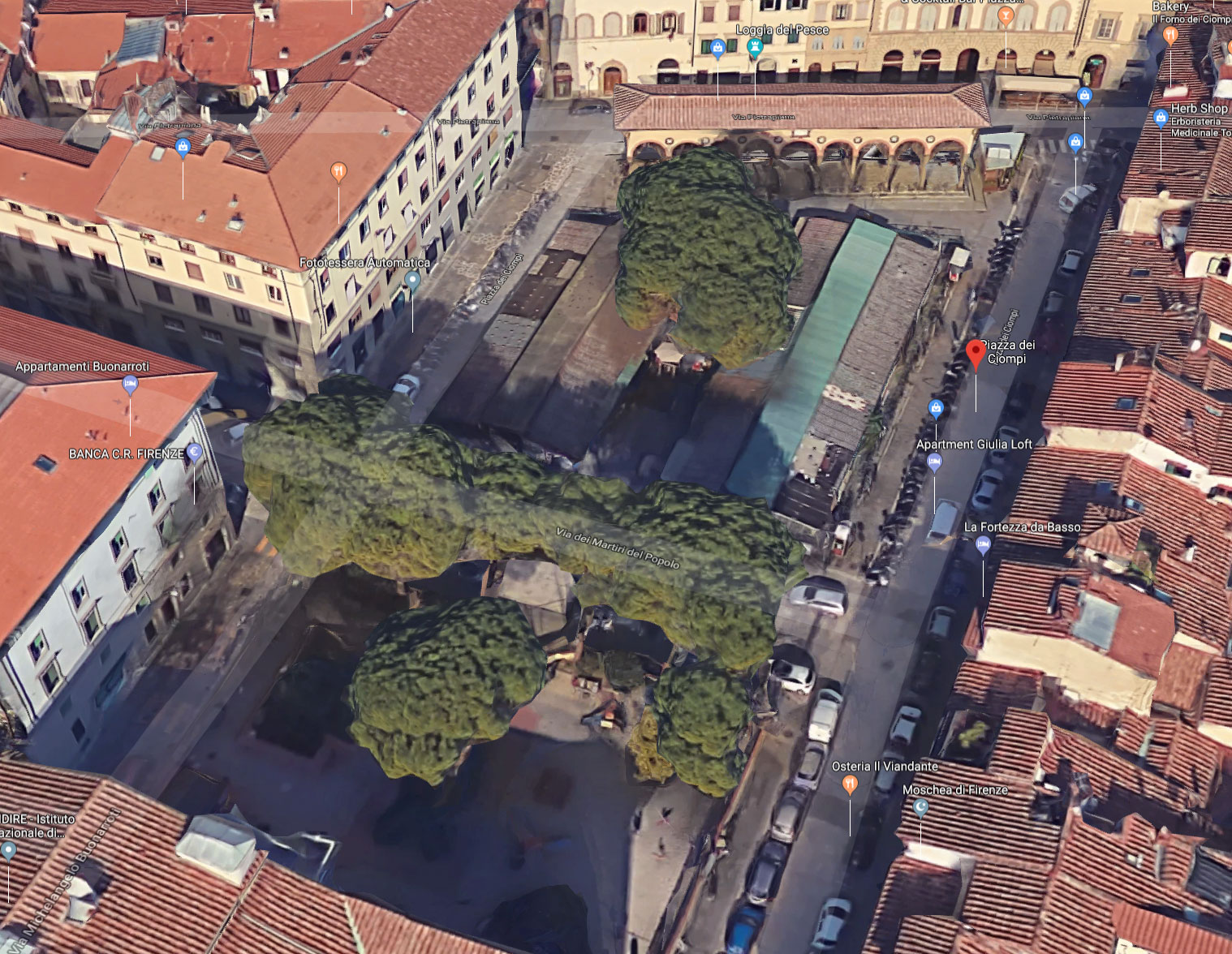This is a top-down, bird's-eye view of a city block likely taken from Google Maps. The image showcases a central open area with some trees and a cement section, possibly functioning as a small park or plaza. Surrounding this open space are multiple buildings exhibiting distinct European architecture, strongly suggesting that the location is in Italy, possibly based on the street names and specific labels such as "Piazza de Chiompi" and "Banca Firenze."

The buildings include a mix of residential units with rooftop gardens and patios, as well as single-type homes. There are various points of interest such as apartments, restaurants, and hotels identified in the image. The streets are bustling with vehicles, highlighting the urban setting. Additionally, the top of the image shows what might be repurposed stalls, hinting at a former bus or carriage station. The presence of several cars parked along the streets emphasizes the active, lived-in nature of this Italian locale.